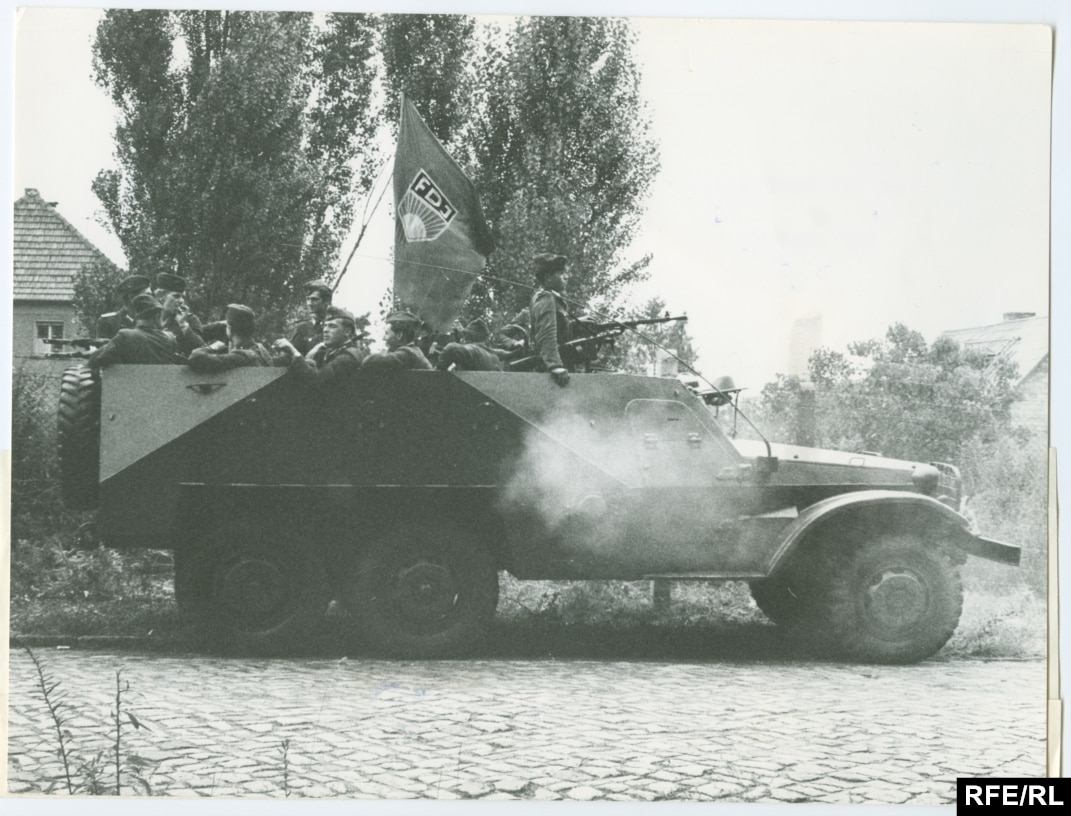This black-and-white photograph, marked "RFE/RL" in the bottom right corner, captures a wartime scene with striking detail. The image features a large, open-top tank truck navigating a cobblestone road, surrounded by a fog of either smoke or mist. Occupying most of the truck, eleven soldiers in military uniforms, some wearing berets, are visible. One soldier prominently stands at the front with a gun pointed outward, suggesting readiness for combat. The presence of gun smoke indicates possible recent shots fired. The tank truck is moving forward, towards the right, with three large wheels distinctly visible – one in the front and two in the back. In the distant background, there are trees and buildings, implying an urban setting. A flag bearing the letters "FDJ" flutters on the vehicle, though its significance remains unclear. The bottom left corner of the image shows some foliage intruding into the frame, adding a touch of nature to the otherwise stark wartime environment. The overall atmosphere, combined with the soldiers’ postures and the surrounding elements, evokes a vivid sense of historical conflict, possibly from World War I or II.